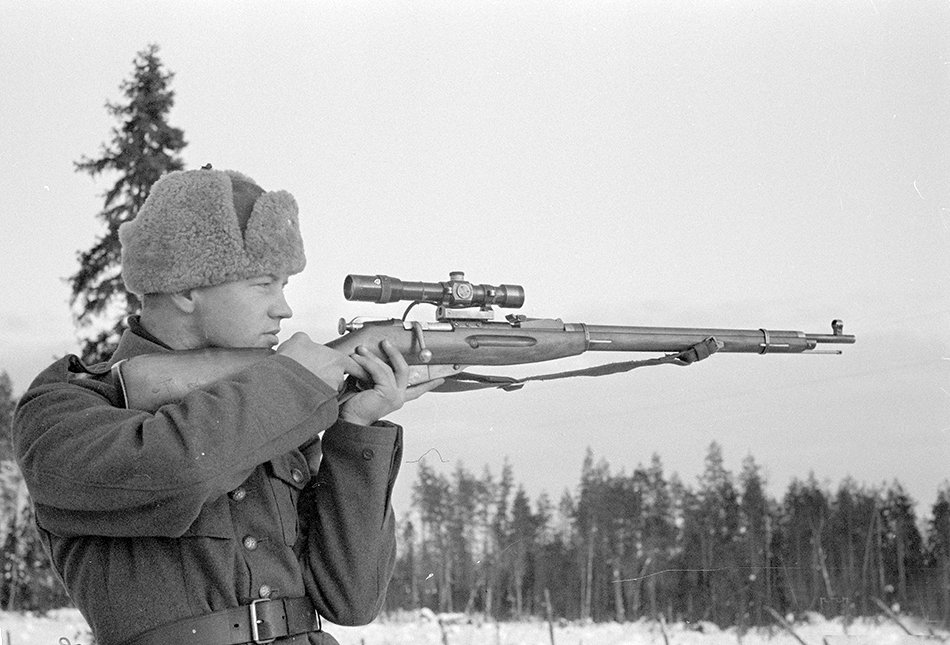This is a detailed black and white photograph capturing a wintry scene. The day appears overcast, with a white sky contrasting against a backdrop of dark pine trees and a barbed wire fence. Snow blankets the ground. On the left side of the image, a man with a fur hat that has folded-up wool on the sides stands in profile, facing to the right. He is wearing what looks to be a 1940s-era military uniform, complete with a black wool coat, buttons running down the front, a comically oversized black leather belt with a buckle, and no visible badges or patches. Cradled in both hands, he holds a long, bolt-action rifle equipped with a scope. He appears to be just starting to look into the scope, but not directly through it. The photograph, wider than it is tall, hints at a historical setting, possibly involving a Russian sniper, though no text or date indicates the precise time period captured.